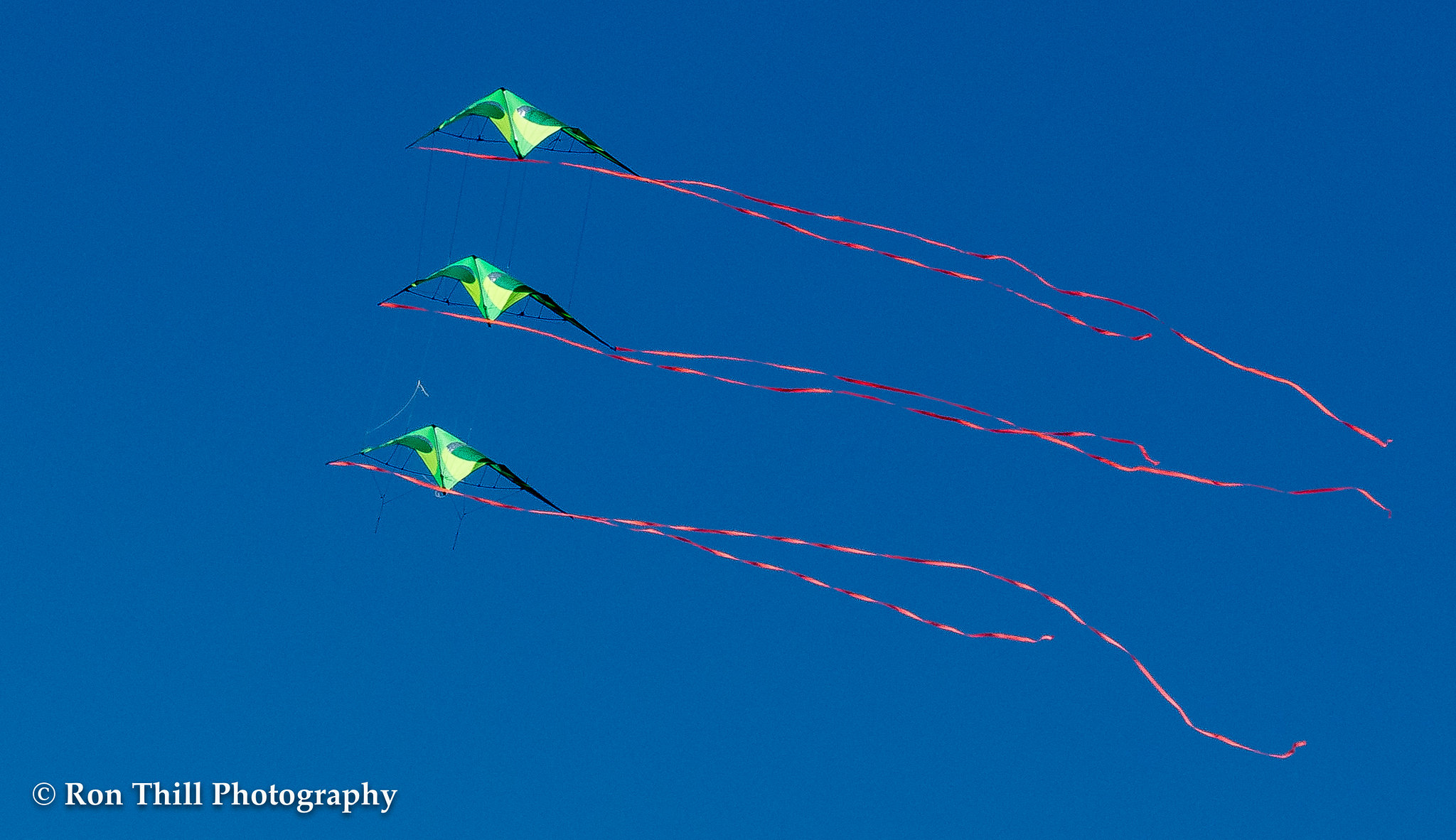This landscape-oriented photograph, credited to Ron Thill Photography in white letters at the bottom left corner, captures a vivid scene of three visually identical kites flying in a deep, even medium-blue sky. Each kite features a green, diamond-shaped design with varying shades of green; a lighter green center contrasts with darker green tips, accented by almost eye-like patterns near the top. The kites, seemingly individual at first glance, are actually connected by barely visible strings, creating a mesmerizing vertical alignment. Trailing from each kite are two red streamers, shimmering in shades from light pink to deep red, gracefully flowing to the right, adding a dynamic sense of movement to the serene sky. Together, these elements form a striking display of three green diamonds and six vibrant red ribbons dancing in perfect harmony.